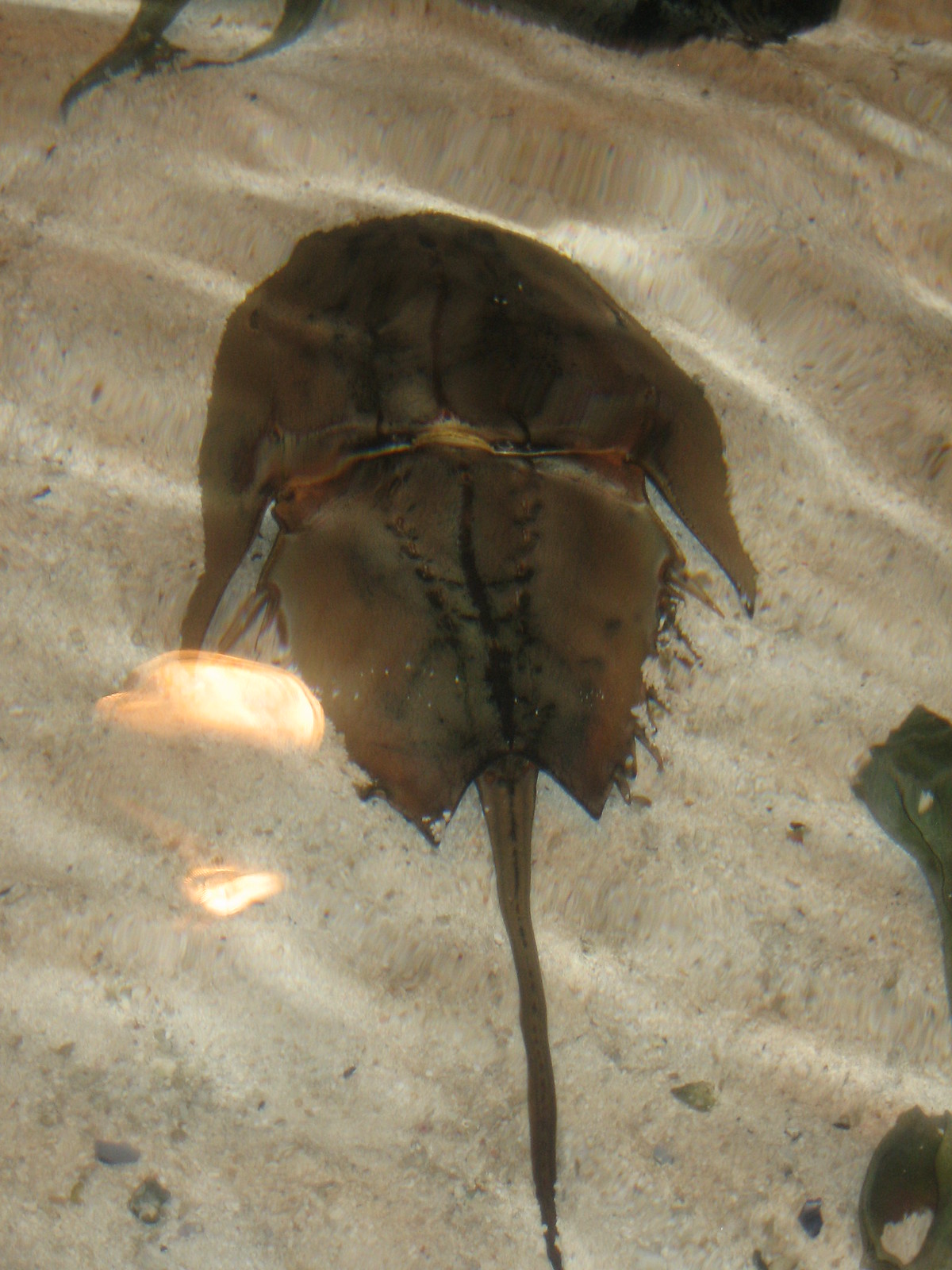This is a vertically aligned rectangular image depicting an aquatic animal, most likely a brown stingray, submerged underwater. The stingray exhibits a wide, circular body adorned with distinct black lines, and its long, thin brown tail extends downward toward the bottom of the picture. The surrounding environment resembles a sandy floor scattered with small rocks, suggesting the photo might have been taken in a shallow beach area or an aquarium enclosure. There are light reflections on the water's surface, adding a shimmering effect to the scene. In the image's upper left corner, part of another aquatic creature's tail can be seen, hinting at the presence of more marine life outside the main frame. Additionally, the right edge of the image shows a portion of another brown object, possibly another animal. The overall lighting suggests that the image might have been taken in a dim setting, either at night or in a darkened aquarium exhibit.